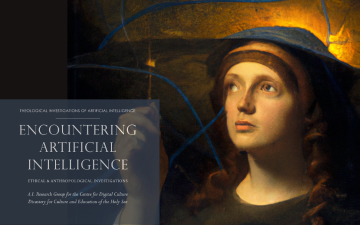The image is a digital and painting hybrid, set in a horizontally rectangular frame with no definitive border or background. Dominating the right side is a woman with fair skin and curly brown hair falling just below her shoulders. She is dressed in a blue robe with a hood covering her head and is intently looking towards the upper left-hand corner of the picture. In her hand, she holds a small, thin object which could be a match or a key. Behind her, there is a warm, yellowish glow, possibly indicative of the sun. The lower left corner features a transparent navy blue box containing white text. The most legible part of the text reads "Encountering Artificial Intelligence," followed by smaller sentences and a paragraph that are too small to decipher. The background of the image transitions from brown to blue with decorative lines, adding a layered, artistic touch to the scene. This image appears to be a cover for a presentation, course, or book on the topic of artificial intelligence from an ethical and investigative perspective.